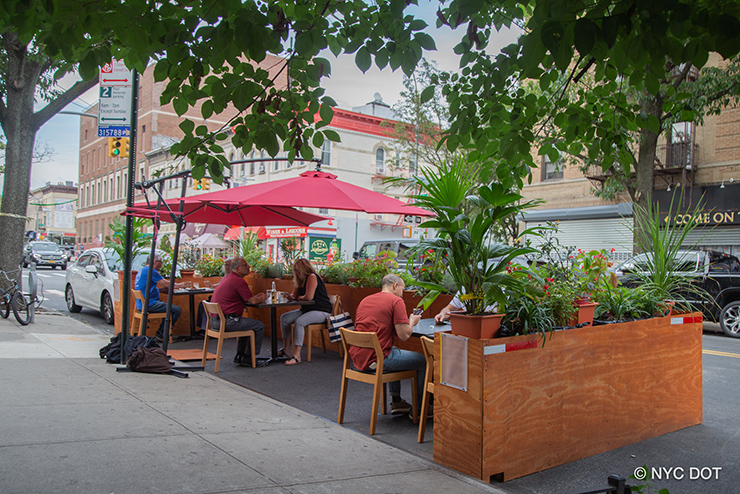This is a vibrant, sunny daytime city street scene featuring an outdoor dining area that occupies a section of the street typically reserved for cars. This makeshift seating area, attached to a cafe or restaurant, is thoughtfully partitioned with wooden panels adorned with various plants, including green flowers and palm trees. The area consists of four small tables, each paired with two chairs, all of which are occupied. People at the tables are engaged in conversations or perusing menus; notably, one woman has a black and white Sephora bag hanging off her chair. Red umbrellas provide shade over the diners. Surrounding the dining area, there's a mix of parked and moving cars, a bus sign pole, and a large tree with a bicycle on the sidewalk. Across the street, various businesses with storefronts line the bottom of large buildings. At the bottom right corner of the photo, the text “NYC dot” is visible within a white circle.